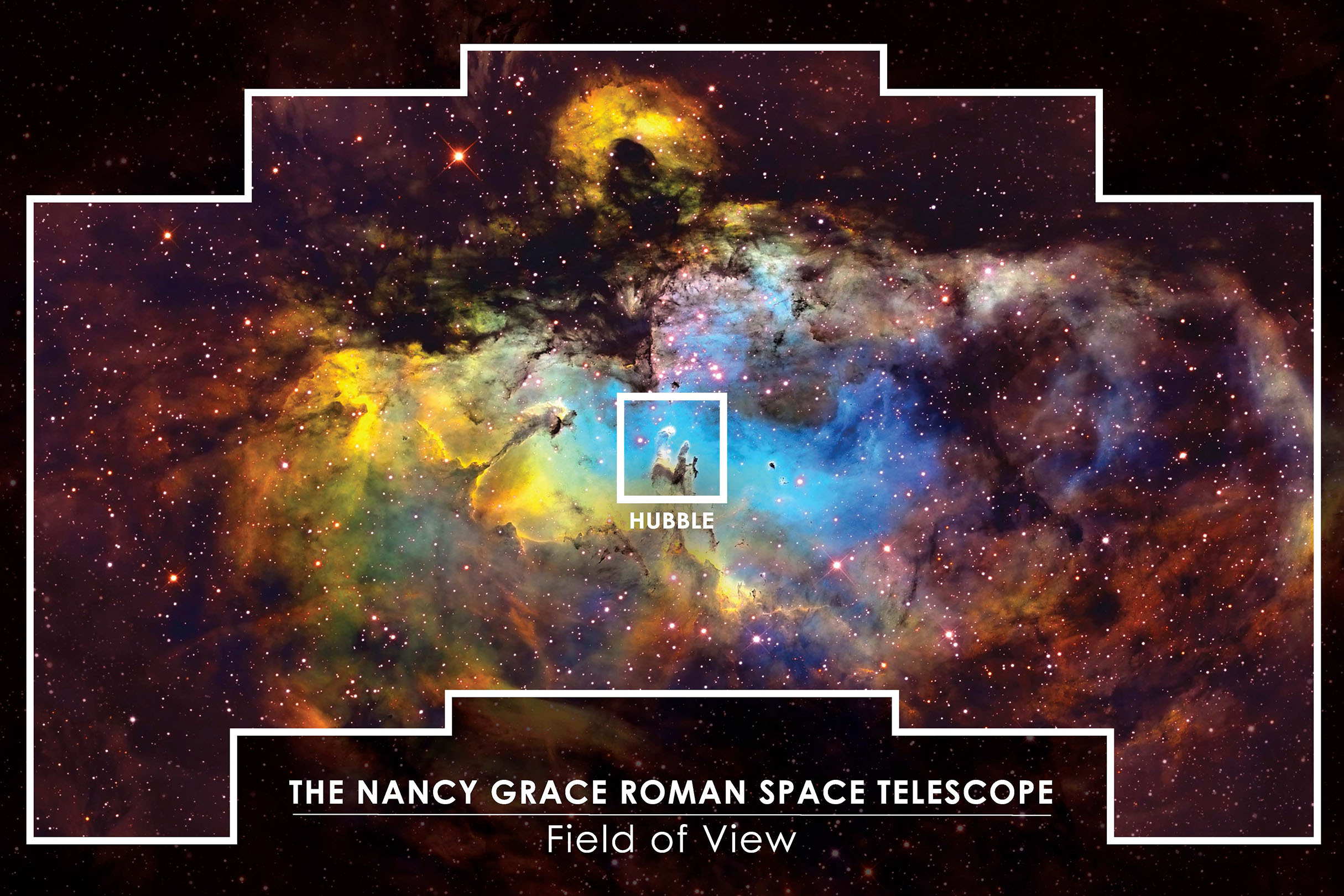This image, presented in a landscape layout with a black background, features a detailed, colorful view of outer space. Along the bottom of the image, centered in bold, all-capital white text, are the words "THE NANCY GRACE ROMAN SPACE TELESCOPE," with a line underneath. Below this line, also centered but in non-bold white text, it reads "Field of View." Above this text area is a prominently outlined irregular white border, representing a section of space. Inside this border, the black space background is richly dotted with small pink, yellow, and red stars, along with vibrant hues of blue, purple, yellow, orange, and green clouds intermingling. 

At the very center of the image, another white square outline encloses a similar colorful space segment labeled "HUBBLE," also in bold, capital white letters. This central area specifically highlights hues of blues, whites, and pink dots, indicating a different field of view within the broader panorama. The entire image depicts a visually stunning and intricate cosmic landscape, showcasing a myriad of colors reminiscent of all the hues of the rainbow amidst the vast darkness of space.